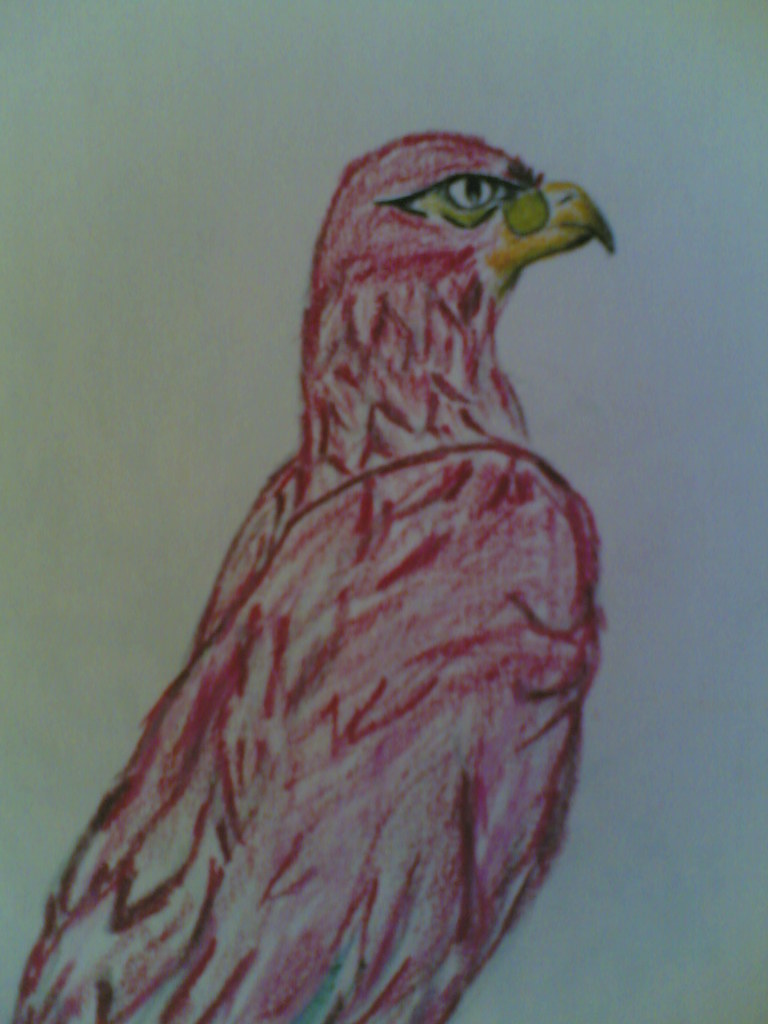This is an illustrative image set against a white background, depicting a bird in striking pink and red hues. The bird is positioned in a proud and assertive stance, showing a side profile while perched and gazing towards the right. Its chest is prominently puffed out and its head held high, exuding an air of strength and pride. The bird features a yellow beak accentuated with strong black line work at the edges, culminating in subtle black shading at the tip. Its eyes are expressive, with a black pupil set against a white background, encircled by a green area that adds depth. The eyes are further defined by additional black line work, creating an impression of a secondary eye shape. The bird's feathers showcase a gradient from pink to darker red, meticulously outlined to highlight each feather with precision.